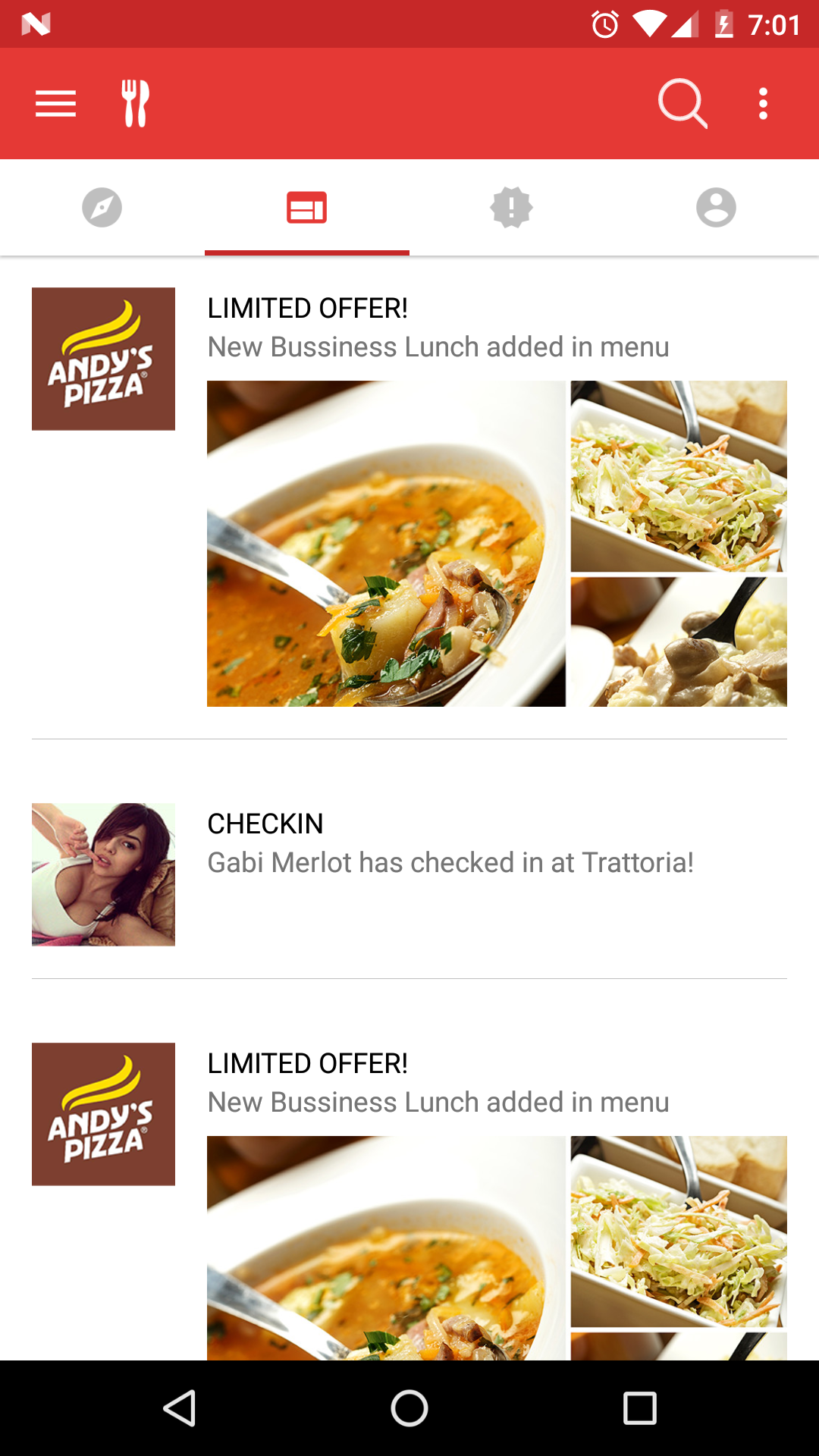### Detailed Caption for Andy's Pizza Ad on Mobile

This advertisement from Andy's Pizza is displayed on a mobile phone screen. The top section of the ad features a red header with a maroon stripe, inclusive of a search bar on the right side that is adorned with a knife and fork icon, alongside a menu drop-down option. The phone's default icons, such as battery life and signal strength, are visible at the very top.

Moving down the ad, there's a highlighted section beneath the red header showcasing various offers. The prominent banner on the left-hand side displays Andy's Pizza logo, a brown square sign with yellow squiggles at the top and the text "Andy's Pizza" in the center.

A noteworthy promotion is detailed in the ad. There's a special notice of a "limited offer" for a new business lunch addition to the menu. The visual focus includes a large image of soup, indicating that Andy's Pizza serves more than just pizza. Accompanying this image are two smaller pictures: one of coleslaw and another dish that appears to consist of meat and noodles, although exact identification is unclear.

Embedded within the advertisement is a pop-up notification stating, "Check-in: Gabby Merlot has checked in at Trattoria." This pop-up includes a seductive image of a woman with brown hair lying on her side.

Towards the bottom of the ad, the limited offer notice is repeated. The footer of the ad features a black strip containing navigation icons: an arrow pointing left, a circle, and a square.